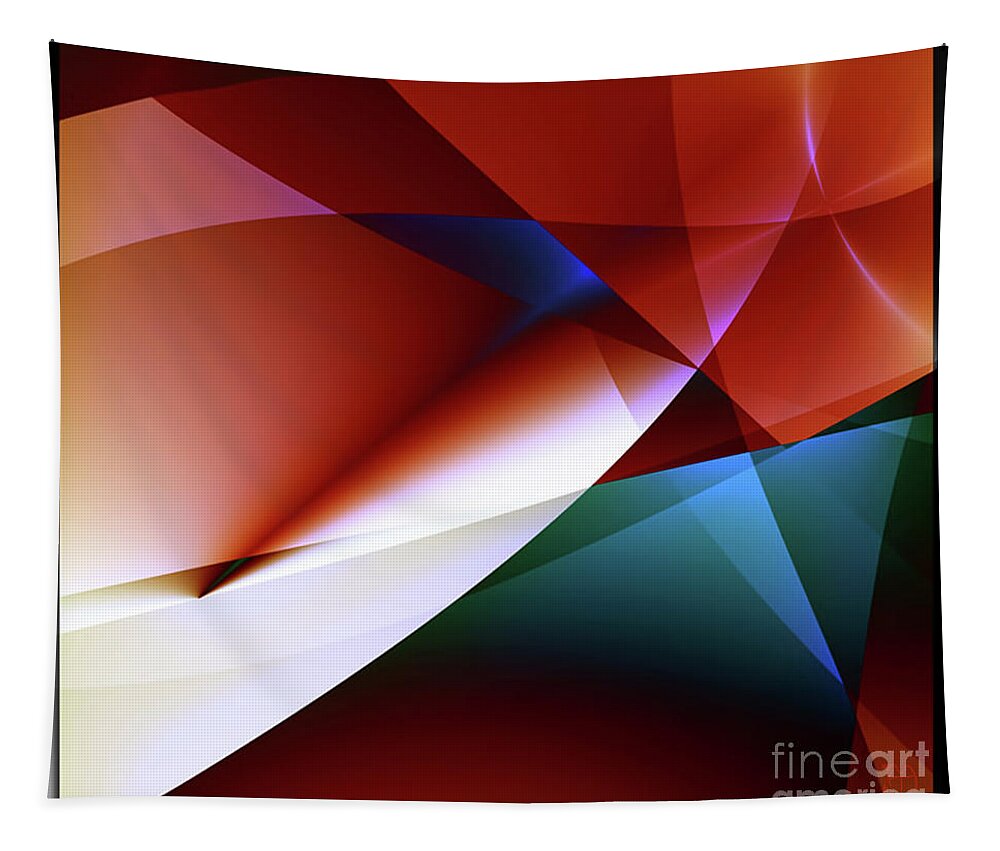This is a color image of an abstract, computer-generated graphic design. The central decoration spans the entire composition and consists of translucent, overlapping geometric shapes with curved edges, including triangles, bands, and other forms. These shapes display a variety of colors such as red, blue, green, light blue, light purple, and white, creating a layered, intricate pattern. The top of the image features a sagging blue triangle, while the upper right is predominantly red with pink highlights. The bottom left shows shades of turquoise and light blue, and the bottom edge, especially the lower right, is dominated by dark red and black hues. White lines and white portions also contribute to the overall design. The entire piece, which appears to sag at the top and curve on the sides, resembles a fabric hanging on a wall against a white background. In light gray text at the lower right corner, there is a watermark that reads "Fine Art America," although the word "America" is partially cutoff.